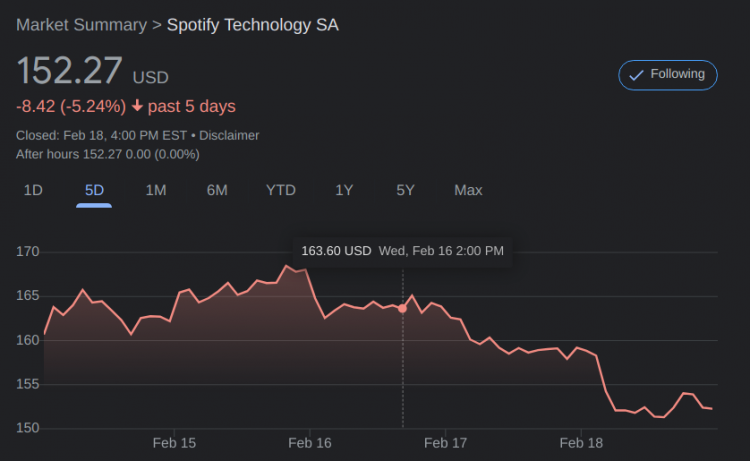This screenshot displays a stock market summary for Spotify Technology SA on a computer screen with a black background. The title "Market Summary" is prominently displayed at the top in white letters, followed by "Spotify Technology SA" in slightly brighter white text. The current stock price is shown as $152.27 USD in gray letters, accompanied by a red indicator of recent performance: "-8.42 (-5.24%)" with a downward arrow, signifying a decline over the past five days.

Additional details, such as the market status indicating "Closed," include the date, time, and a disclaimer. "After Hours" information is also present in this section. Below this summary, a detailed line graph illustrates the stock's performance. The top of the graph features selectable time ranges including 1 day, 5 day, 1 month, 6 month, year to date, 1 year, 5 year, and max.

The vertical axis of the graph is labeled with stock prices ranging from $150 to $170 in $5 increments, while the horizontal axis is marked with dates: February 15th, 16th, 17th, and 18th. The line graph itself is jagged with numerous fluctuations, depicted in a reddish color with a slightly shaded reddish-orange area beneath it. An intersecting line highlights a specific point where the stock was valued at $163.60 USD on February 16th at 2 PM.